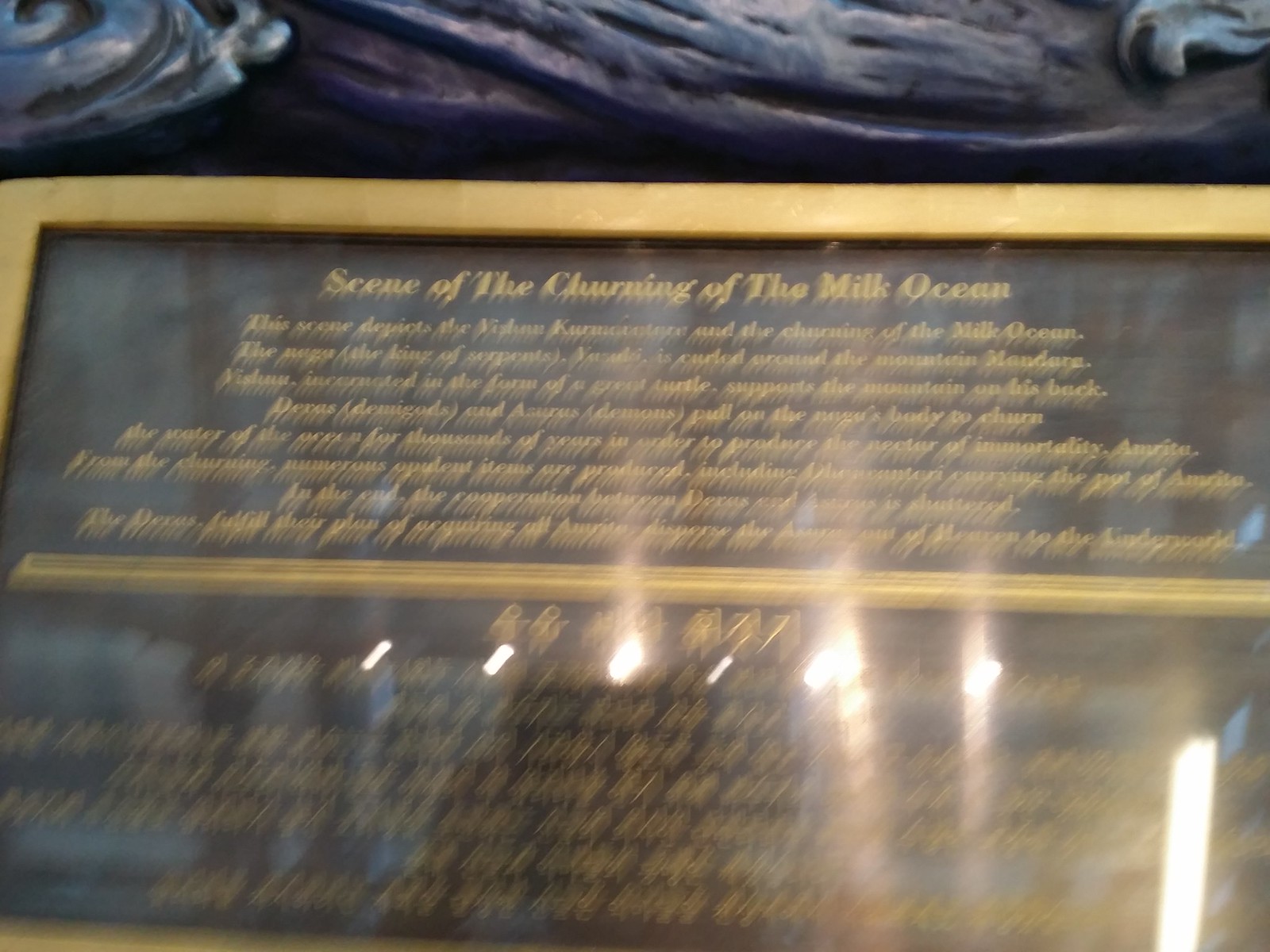The image is a rectangular, low-resolution and blurry photograph that appears to capture an item in motion. The central subject of the photo seems to be a square-shaped object. This object has a golden border at the top, with a predominantly black background. Within the square, there are two blocks of text: the one at the top is in English and reads, "Scene of the churning of the milk," while the one at the bottom consists of Korean characters. The overall image quality is poor, making the details fuzzy and indistinct.